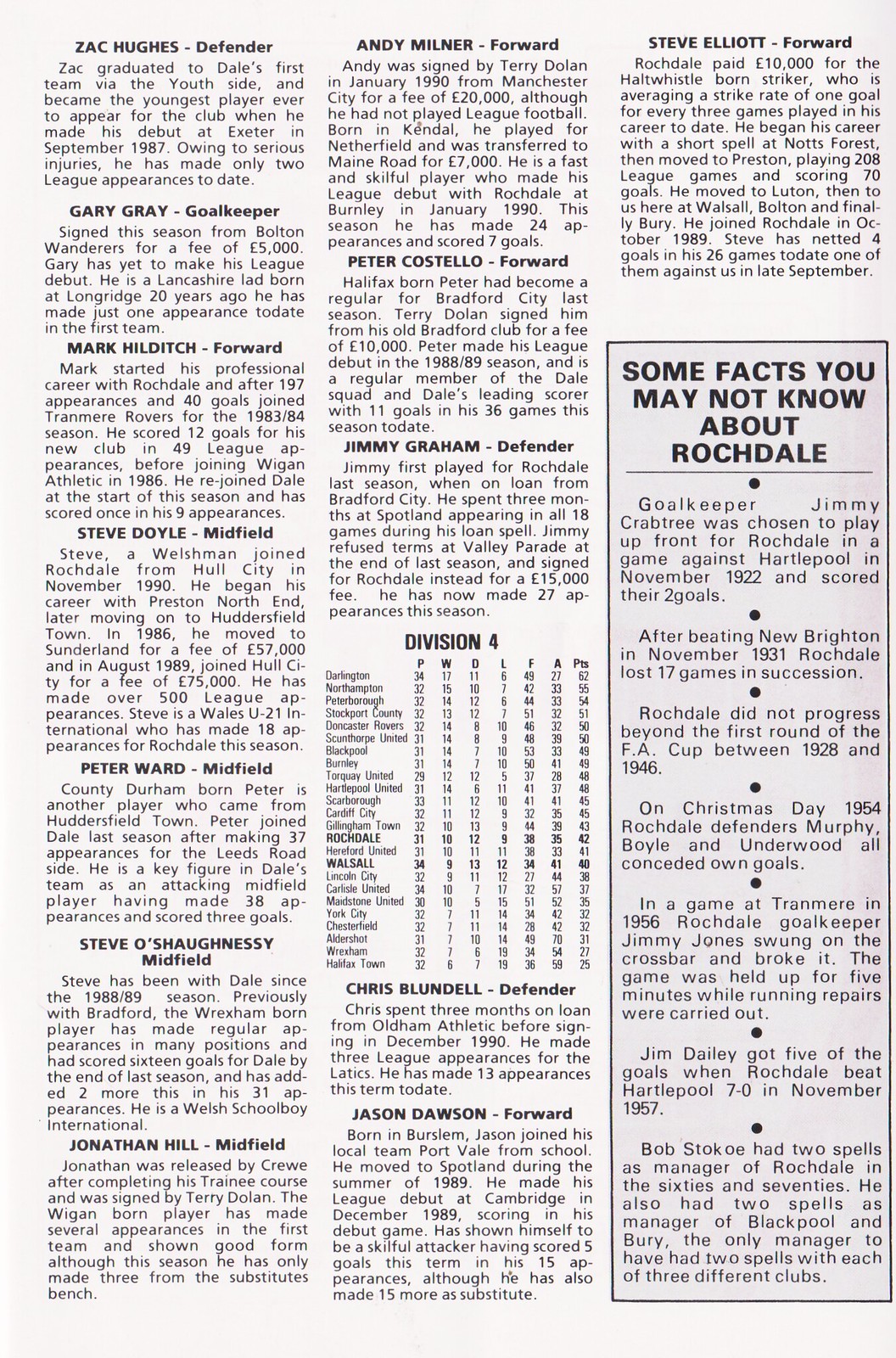This sporting flyer, designed like a magazine page, features detailed bios of various players and is organized into three sections. The first section lists player names and their positions: Zach Hugh (defender), Gary Gray (goalkeeper), Mark Hilditch (forward), Steve Doyle (midfield), Peter Ward (midfield), Steve O'Shaughnessy (midfield), and Jonathan Hill (midfield). The middle section continues with more players and their biographies, including D. Milner (forward), Peter Costello (forward), Jimmy Graham (defender), Chris Blundell (defender), Jason Dawson (forward), and Steve Elliott (forward). The final section presents interesting facts about Rochdale, highlighted in bullet points and located beneath Steve Elliott's bio. Also included are additional statistics and details about Division Four teams.